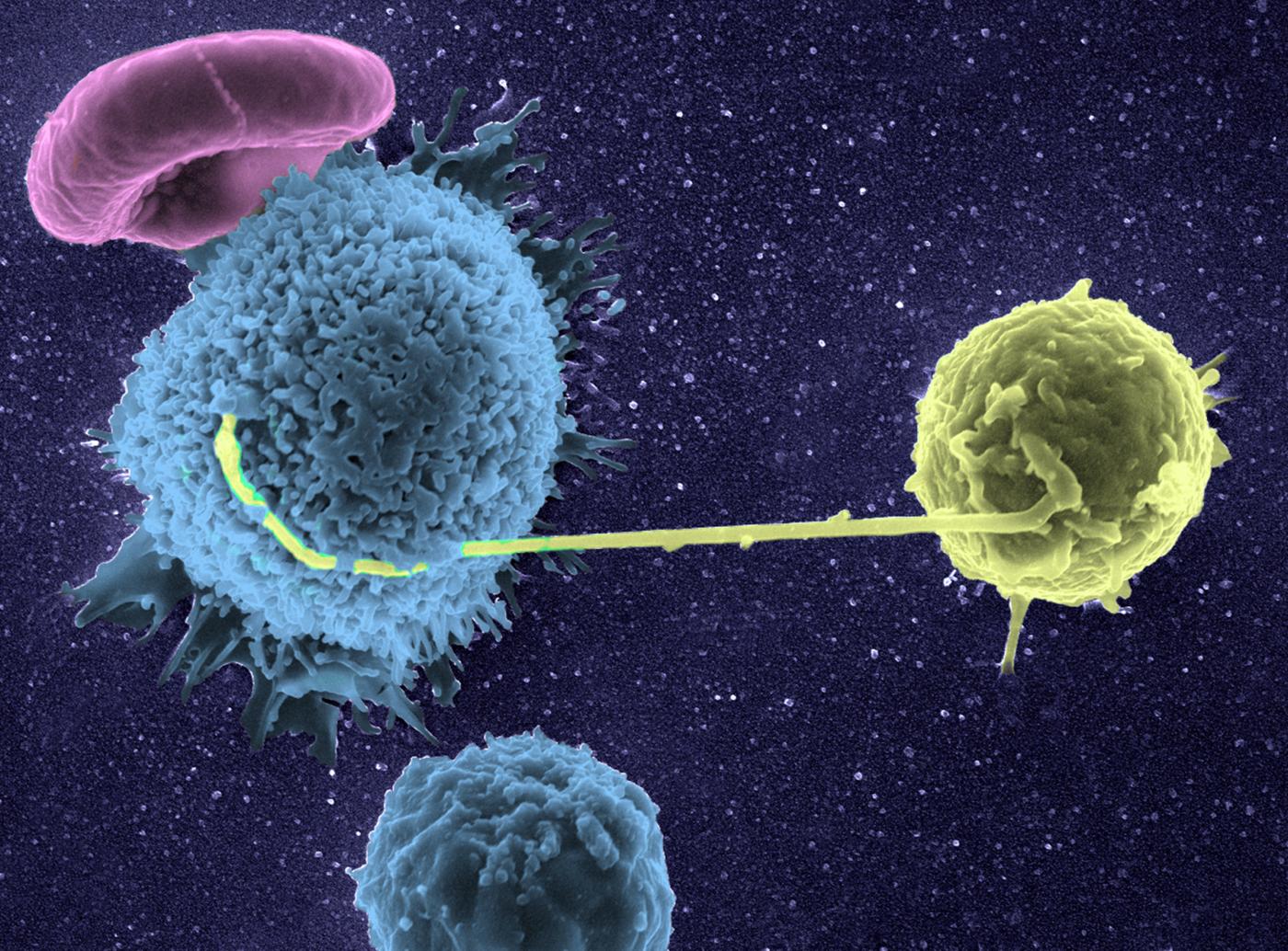This image appears to be a detailed microscopic picture of various cells, set against a background that looks like a deep, dark sky filled with stars, creating a night sky illusion with a purple to black gradient and white star-like dots. In the upper left corner, there is a smooth, pink mushroom cap-like cell with a small stem. Below that on the left side, there's a large, blue, cone-shaped fuzzy cell, and beneath it, a smaller, round blue cell with a bumpy texture. A green line stretches horizontally across the middle of the image, connecting a green fuzzy object on the right side to the aforementioned cells. In the lower left corner, another smaller blue cell is visible. The intricate arrangement of these colorful cells against the starry background creates a surreal, cosmic effect, making the cells appear as though they are floating in space.